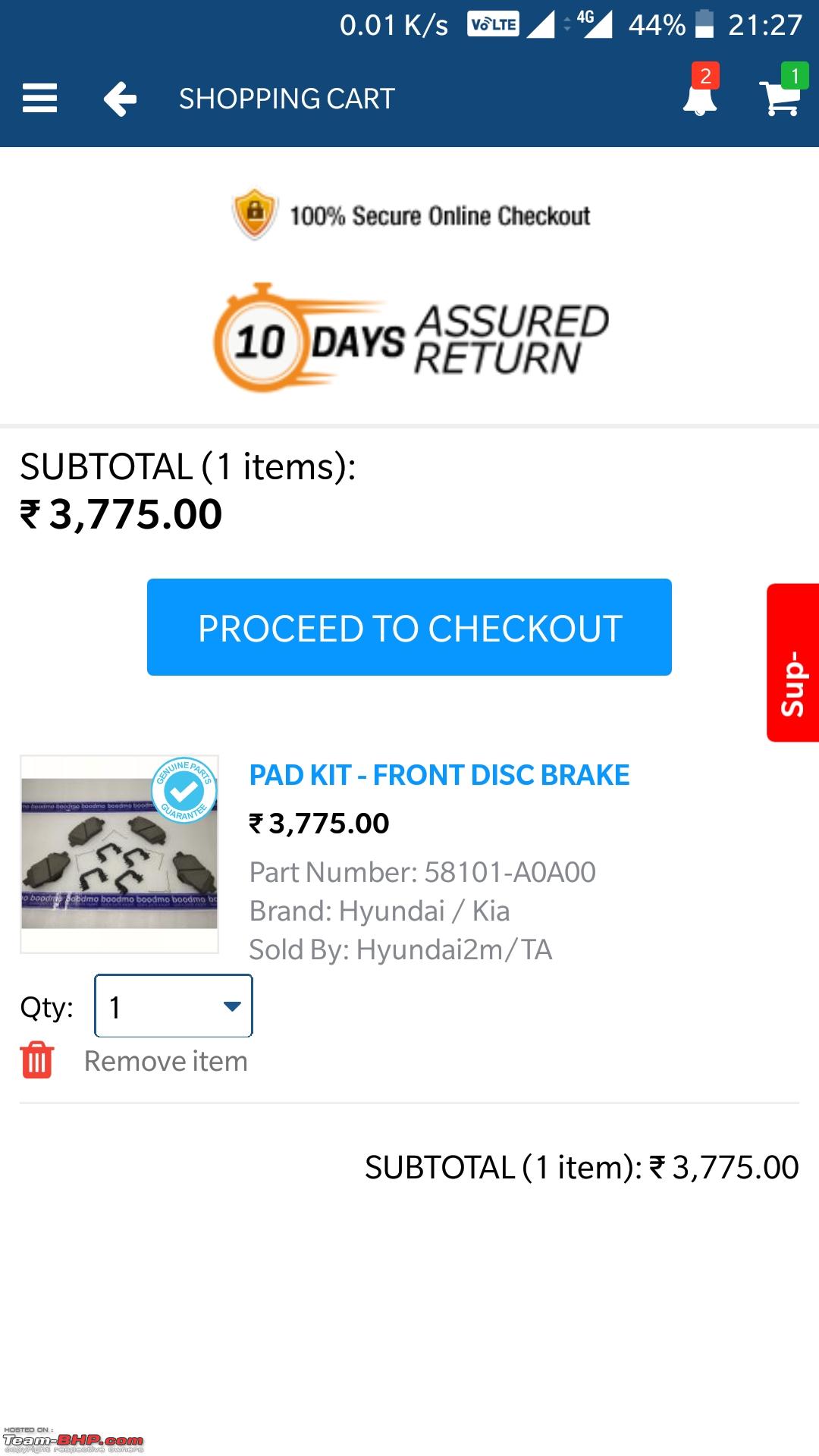A detailed descriptive caption for the image could be:

"This image displays a phone screen with a shopping app open. The status bar at the top reveals various indicators: a signal strength reading of 0.01 K/S, a volt icon, 4G network signal, a secondary network icon, a battery level at 44%, and the time showing as 21:27. Below the status bar, prominently displayed messages assure users of '100% secure online checkout' and '10 days assured return'. The midsection of the screen lists the subtotal for an item, specifically $3,755 for a product identified as a 'Pad Kit, Front Disc Brake,' which is a car part compatible with Hyundai and Kia vehicles. Towards the bottom of the image, icons represent navigation options in the app—an arrow pointing left, a bell icon signaling 2 notifications, and a shopping cart icon showing 1 item. There is also a 'shopping cart' label, indicating the user's current section within the app."